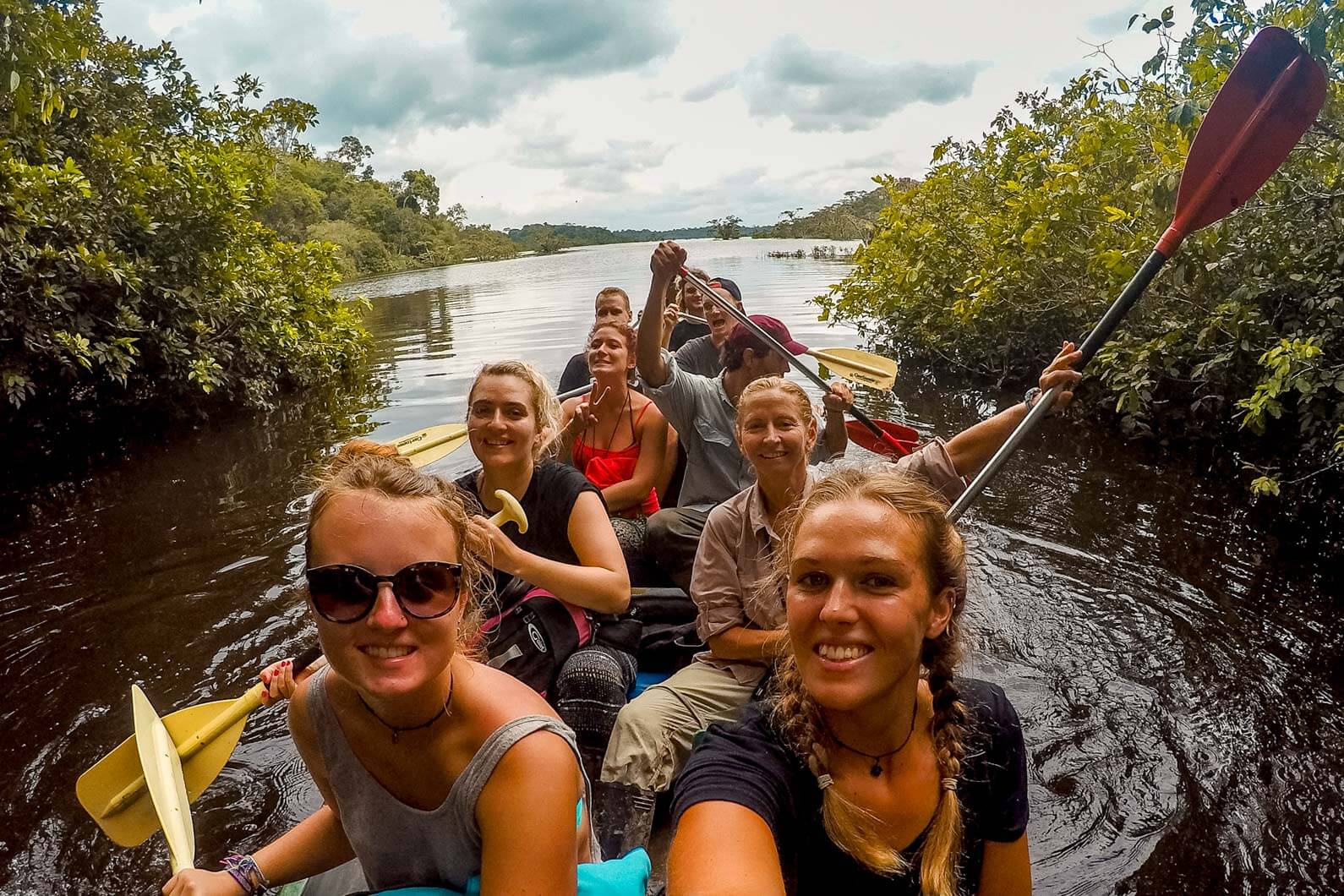The photograph captures a lively group of eight to nine people paddling in either a kayak or canoe through a tropical marshland or river setting. The dark, brackish water contrasts with the lush, green plants hanging over the water's edge on both sides. The sky is a dark blue with heavy clouds, adding to the atmosphere of the scene. At the forefront are two happy, tan, blonde women, one in a gray tank top with sunglasses and another in a short black shirt with braids. Behind them sits another pair of blonde women, one holding a red paddle in the air and another with a paddle dipping into the water. Further back, a woman wearing a red tube top flashes a peace sign while a man beside her, in a short-sleeved button-up shirt, blue jeans, and a red hat, paddles leisurely. Behind them are a few more people, including another man in a blue hat. The overall mood is cheerful, with everyone smiling or engaging playfully, capturing a joyful day out in a scenic, tropical environment.